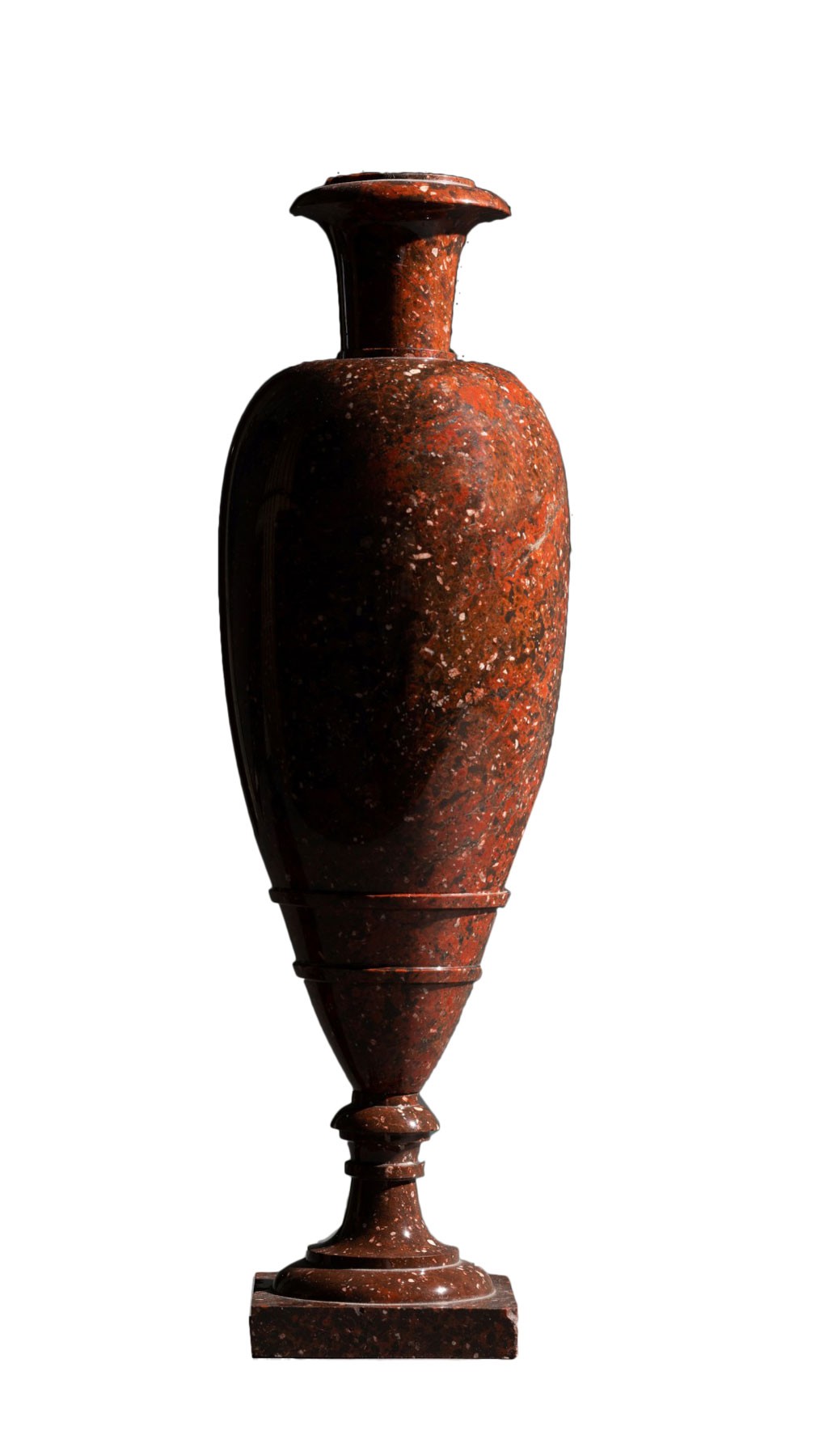This image features a tall brown vessel, potentially a ceramic vase or an umbrella holder, standing against a stark white background. The vase, with a mottled rust color, showcases intricate design details, including speckles of white and black. Its form transitions through various widths: starting at a square base, it leads up to a round disk, then a slightly smaller round disk followed by a cylindrical segment. It then expands into an almost carrot-like or heart-like shape, tapering in at the neck before flaring out towards the middle and narrowing again towards the top, where it opens up. The vessel also features two distinct bands about two-thirds of the way down. One side of the vase is noticeably darker, suggesting a light source from the opposite side, highlighting the object's unique contours and giving it a three-dimensional appearance.